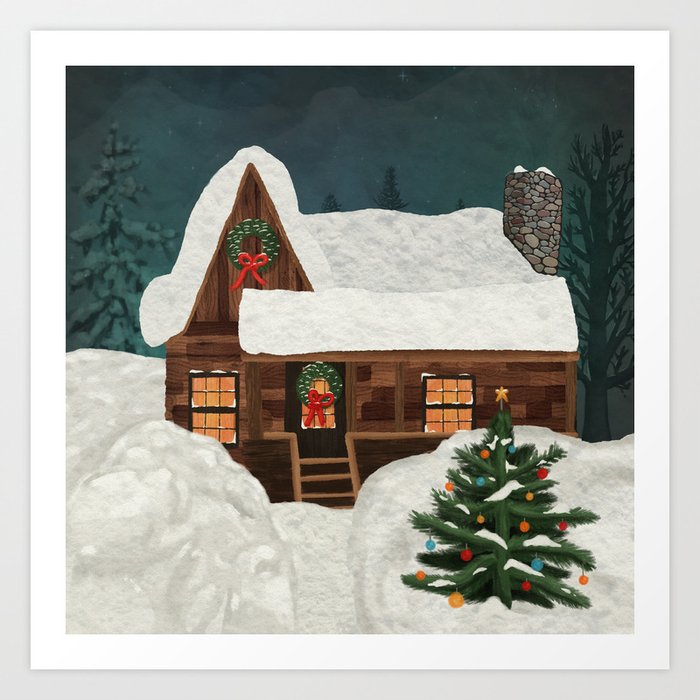The artwork, reminiscent of a Christmas card, captures a serene winter night and depicts a charming brick house enveloped in snow. Set against an off-white wall and framed with a solid white border, the image reveals a cabin with a peaked roof under a starlit sky, subtly strung with blurred stars. The roof is cloaked in snow, with a stone chimney adding to its rustic charm. Atop the roof and on the front door, green wreaths adorned with red bows and lights symbolize holiday cheer. 

In the foreground, two stacks of snow bookend the scene - the left stack stands plain, while the right stack cradles a festively decorated Christmas tree, gleaming with orange, blue, red, and yellow ornaments and crowned with a star. Flanking the house are two pine trees; the left one is heavily laden with snow, whereas the right stands bare. Illuminated windows cast a warm, yellow-orange glow from within, hinting at life and coziness inside. The house entrance, accessible by a few snow-laden stairs, completes the inviting winter tableau, all presented in an artistic style that mimics a collage of stacked paper layers.